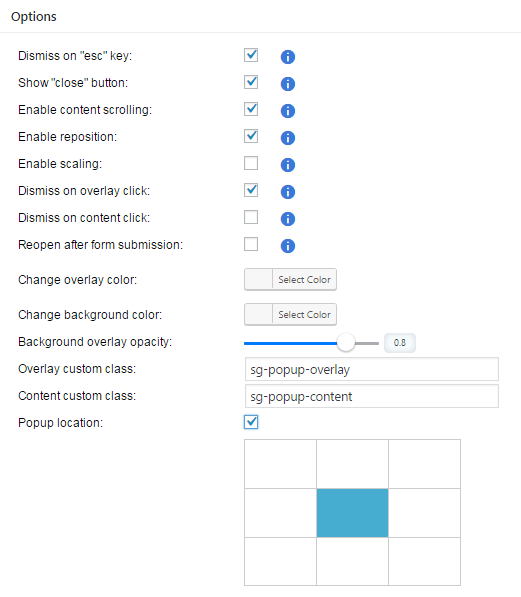This image is a detailed screenshot of an options menu from an unknown application or software interface. At the top, the heading reads "Options."

1. **Dismiss on ESC key**: A checkbox labeled "Dismiss on ESC key" is checked. Accompanying this option is a blue circle with a white eye icon indicating additional information.
2. **Show close button**: This option is also checked, with the information icon next to it for further details.
3. **Enable content scrolling**: The checkbox for this feature is checked.
4. **Enable reposition**: This option's checkbox is checked.
5. **Enable scaling**: The checkbox is checked for enabling scaling.
6. **Dismiss on overlay click**: This checkbox is checked.
7. **Dismiss on content click**: This option is not checked.
8. **Reopen after form submission**: The checkbox for this option is not checked.
9. **Change overlay color**: There is a selectable bar to the right of this option labeled "Select Color."
10. **Change background color**: Similar to the overlay color option, there is a selectable bar to the right also labeled "Select Color."
11. **Background overlay opacity**: This option includes a slider bar set to 0.8.
12. **Overlay custom class**: The field is filled in with "SG-popup-overlay."
13. **Content custom class**: The field is filled in with "SG-popup-content."
14. **Popup location**: A checkbox is labeled here, and at the bottom of the image, there is a rectangular grid made up of nine smaller squares. Only the center square is turquoise blue, while the rest are white, indicating the selected position within the grid for the popup.

This comprehensive screenshot captures a multitude of interface configuration options, visually summarized with accompanying text, icons, and input elements such as checkboxes and sliders.